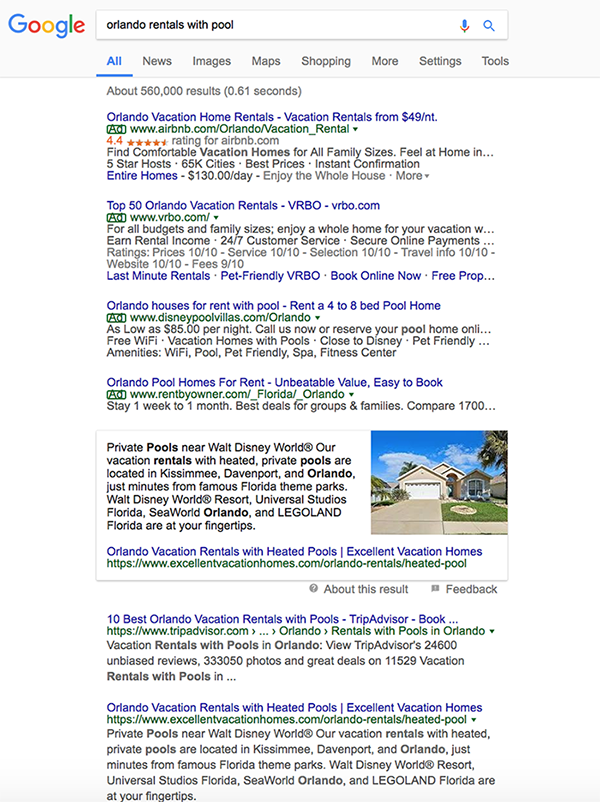The image features a Google search results page with the query "Orlando rentals with pool" entered in the search bar at the top left, accompanied by the Google logo. The search yields approximately 560,000 results in 0.61 seconds.

Highlighted is a search result for "Orlando vacation home rentals" priced at $49 per night through Airbnb. The listing, accessible at "Airbnb.com," boasts a rating of 4.4 stars and offers comfortable vacation homes suitable for all family sizes, hosted by five-star hosts across 65,000 cities globally. Additional features include the best prices, instant confirmation, and the availability of entire homes at a higher rate of $130 per day. The listing encourages enjoying the full house for your stay.

Another prominent listing from "vrbo.com" showcases the "Top 50 Orlando vacation rentals," catering to all budgets and family sizes. This option also features entire homes for vacation use and mentions benefits such as earning rental income, 24/7 customer service, secure online payments, and excellent ratings for various criteria including price, service, selection, and travel information, each rated 10/10. The website fee is noted at $9/10.

Below these listings, there is an image depicting one of the vacation homes available for rent.